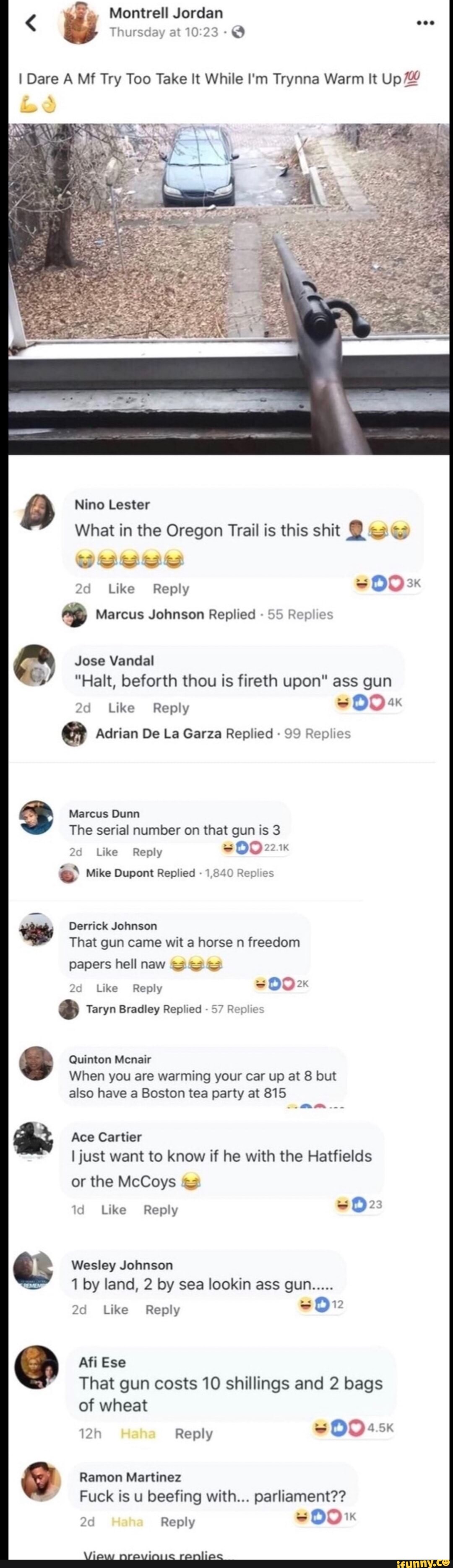This is a detailed and cleaned-up descriptive caption for the given image:

---

This image is a screenshot taken from a mobile phone, capturing a social media post. The post appears to be a response and includes several interactive elements typically found on social media platforms. At the top of the screenshot, there is a faded profile image of a person, making it difficult to discern their features. To the left of the profile image, there is a left-pointing arrow. To the right of the image, the name "Montrell Jordan" is displayed, followed by a timestamp indicating "Thursday at 10:23" along with a globe icon, which usually signifies that the post is public. Further to the right, there are three horizontal dots, commonly representing additional options or settings.

Beneath this header, the main content of Montrell Jordan's post is visible, though specific text details are not provided. The post contains a sentence accompanied by a couple of emojis, suggesting some expression of emotion or context. Additionally, the post includes an embedded media image depicting a scene where a rifle is protruding from a window, seemingly aimed outward. The photograph appears to have been taken during the fall, as indicated by the seasonal elements visible outside. Notably, there are no visible hands holding the rifle, and no person is present inside the car from which the rifle is positioned.

Below the media image, various user profile photos and comments are visible, starting with a comment from "Nino Lester," who remarks, "what’s in the Oregon Trail? Is this shit?" followed by multiple emojis expressing reactions. Each comment has interactive features such as 'like' and 'reply' options, allowing users to engage further with the content.

---

This detailed caption provides a comprehensive description of the screenshot and its elements, making it easier for someone to visualize the content without seeing the image.